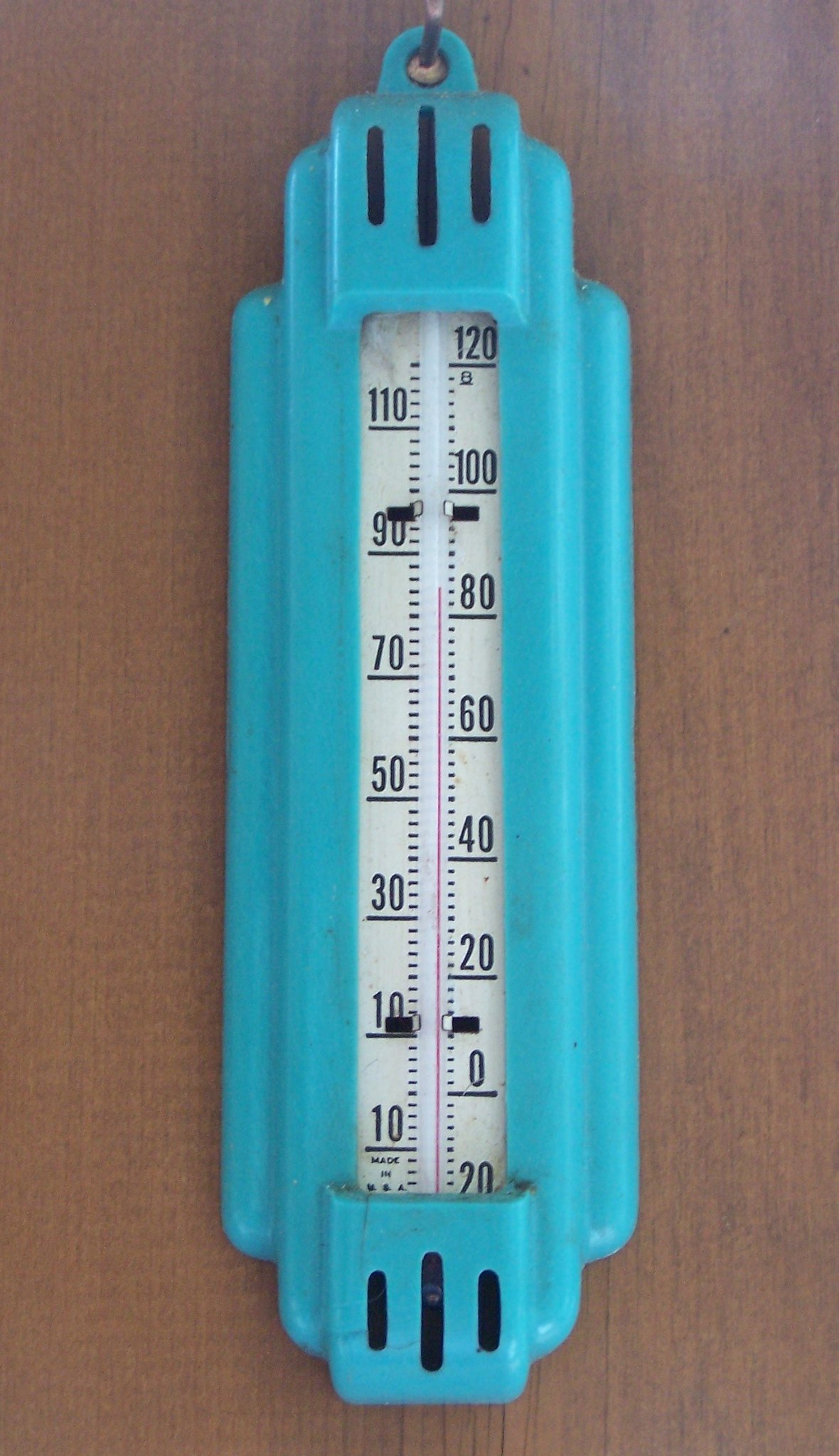This image showcases an outdoor thermometer stylishly encased in a blue plastic housing. The casing features a round loop at the top for convenient hanging, currently suspended from a hook. Below the loop, there's a square segment with three horizontal lines, where the middle line is longer than the two shorter outer lines. The main body extends downward into a longer section, with a similar square and line pattern towards the bottom, mirroring the top design.

In the middle of the casing, there is a white-background thermometer marked with clear numerical increments. On the left side, the temperatures are denoted as 1, 10, 90, 70, 50, 30, 10, and another 10. On the right side, the numbers read 1, 20, 100, 80, 60, 40, 20, zero, and another 20.

The thermometer is mounted against a wooden surface or wall, which has a rich brown color, adding a rustic charm to the overall appearance.